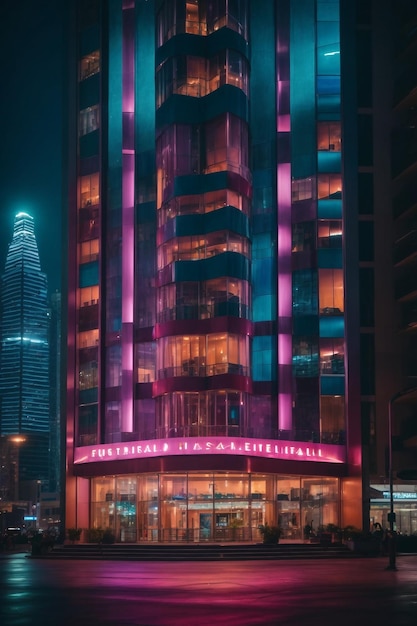The image depicts a vibrant, nighttime cityscape featuring a prominent, tall building in the foreground. This building is strikingly colorful and reflective, adorned with an array of hues including pink, orange, light purple, dark purple, teal, and various shades of blue. Illuminated by these vibrant lights, the structure exudes a powerful presence against the dark sky. The photograph is taken from the street level, looking up at the building, and captures the glow of the lights reflecting off the concrete surface below. There is also text at the bottom of the building, likely in another language, which is blurred and difficult to read. Adjacent to the main building, another taller, blue skyscraper looms in the background, further contributing to the urban landscape. The glass windows of the structures suggest the presence of apartments or condos, enhancing the sense of a bustling city life.